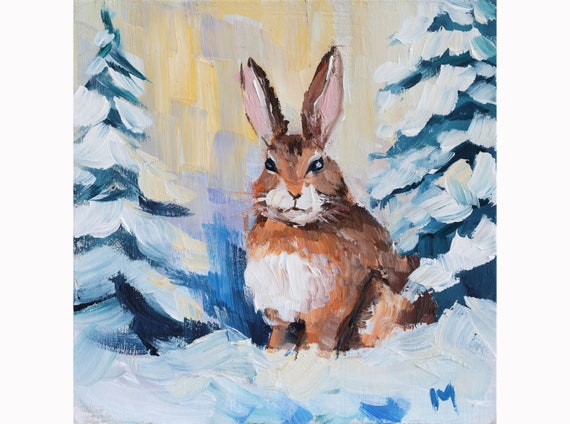The painting depicts a serene, snowy nature scene under a bright sky, transitioning in color from a mix of yellow and purple at the top to dark blue at the bottom. Deep green pine trees, dusted with snow, stand on the left and right sides of the composition, framing the central figure—an endearing brown bunny. The bunny, positioned as the main focal point in the middle of the snow-covered ground, stands with tall, erect ears and is adorned with long whiskers, black eyes featuring white eyebrows, and a white belly that extends to patches around its mouth. The bunny gazes directly at the viewer, creating a captivating and whimsical atmosphere within the wintery landscape.